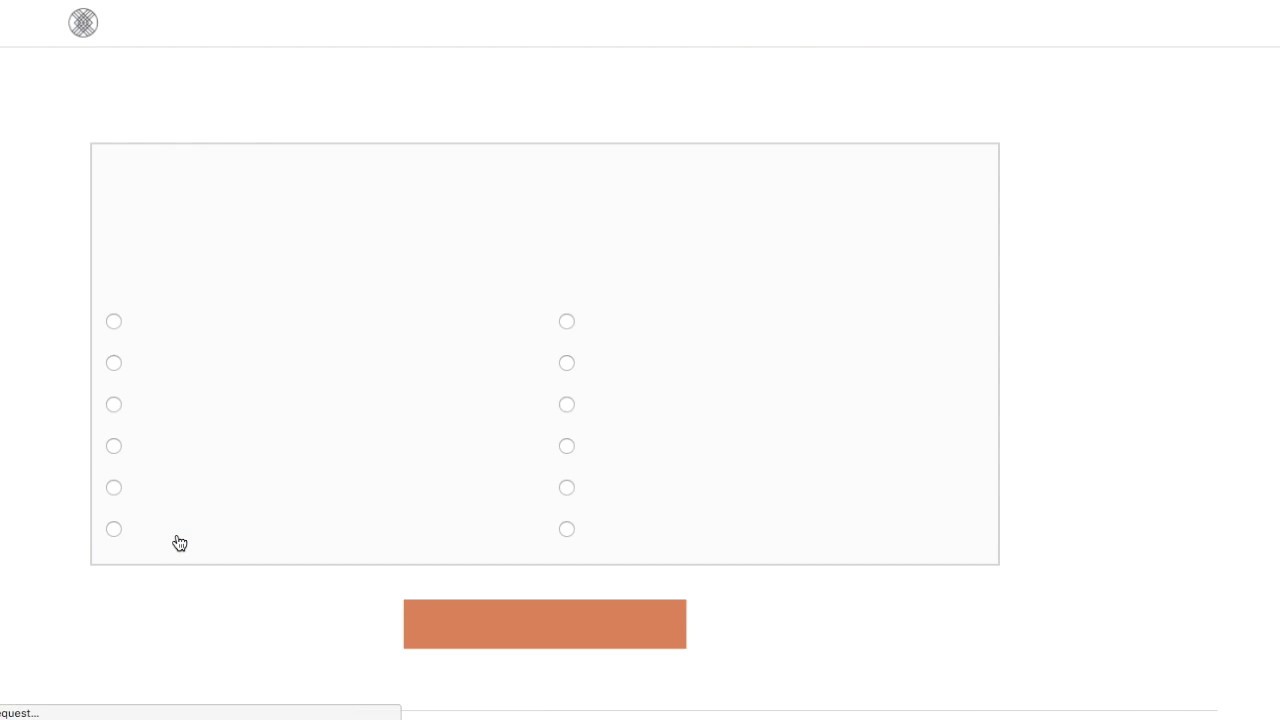The image showcases a user interface likely intended for an online survey, form, or questionnaire. The interface features an orderly arrangement of seven circular buttons organized vertically in the center, split into two columns indicative of possible multiple-choice responses. Dominating the lower portion of the layout is a prominent, yet unlabelled, large orange rectangular button. The interface presents a minimalist aesthetic with a plain white background.

At the top of the interface, a circular icon adorned with a cross is visible, potentially serving as a representational or navigational element. Notably, the screenshot suggests that the form or survey is in an incomplete or unresponsive state, possibly frozen or improperly loaded at the time the image was captured. This could indicate that the screenshot was taken to document a malfunction or issue for troubleshooting purposes, as elements appear unresponsive and no content is visibly loaded within the interface.